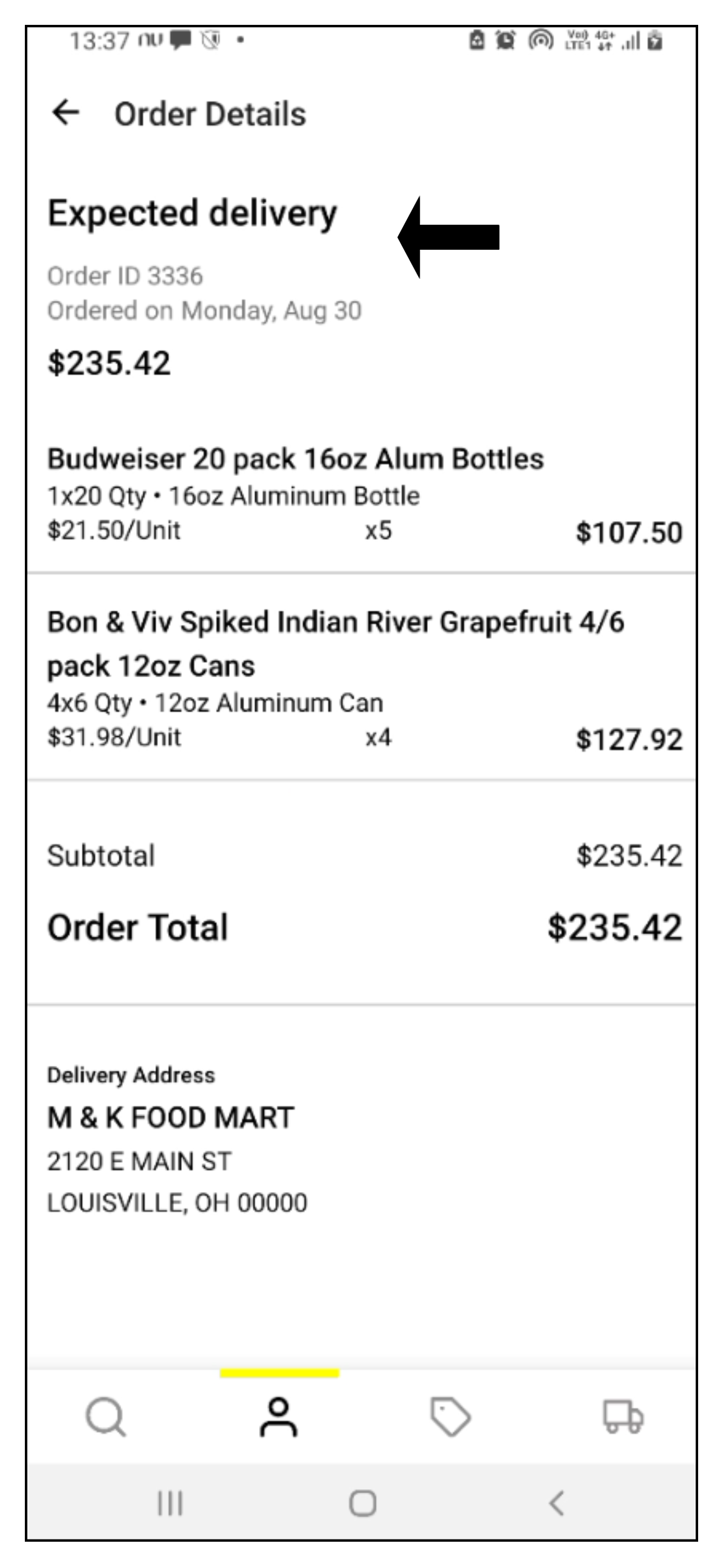This is a screenshot captured on a mobile phone, showcasing a detailed view of an order summary with a white background and black text. At the bottom of the screen, there is a grey navigation bar featuring mobile icons: three vertical lines, a circle, and a back arrow. Just above this, a row of white icons includes a search icon, a person icon with a small yellow line indicating the active tab, a ticket icon, and a van icon.

At the top of the screen, the time displayed is 13:07. On the left-hand side, there are mobile signal and battery icons, while the right-hand side shows a section titled "Order Details" along with a back arrow and an "Expected Delivery" notice. Below this, the order number is partially visible; it appears to be "Order ID 3326" although the text is quite small.

The order was placed on Monday, August 30th, as indicated by a prominent black arrow that seems superimposed over the image. The order's total value is $235.42 and it includes the following items:

1. **Budweiser 20-pack (16 oz aluminum bottles)**:
   - Quantity: 1 pack of 20 bottles
   - Unit Price: $21.50 per pack
   - Total: $107.50

2. **Bon & Viv Spiked Indian River Grapefruit 4/6-pack (12 oz cans)**:
   - Quantity: 4 packs of 6 cans each
   - Unit Price: $31.96 per pack
   - Total: $127.92

The subtotal for the order is $235.42, and this is also the final order total.

The delivery address provided is:
MK Food Mart,
2120 E Main Street,
Louisville, OH 00000.

All these details are carefully laid out, providing a comprehensive snapshot of the placed order.